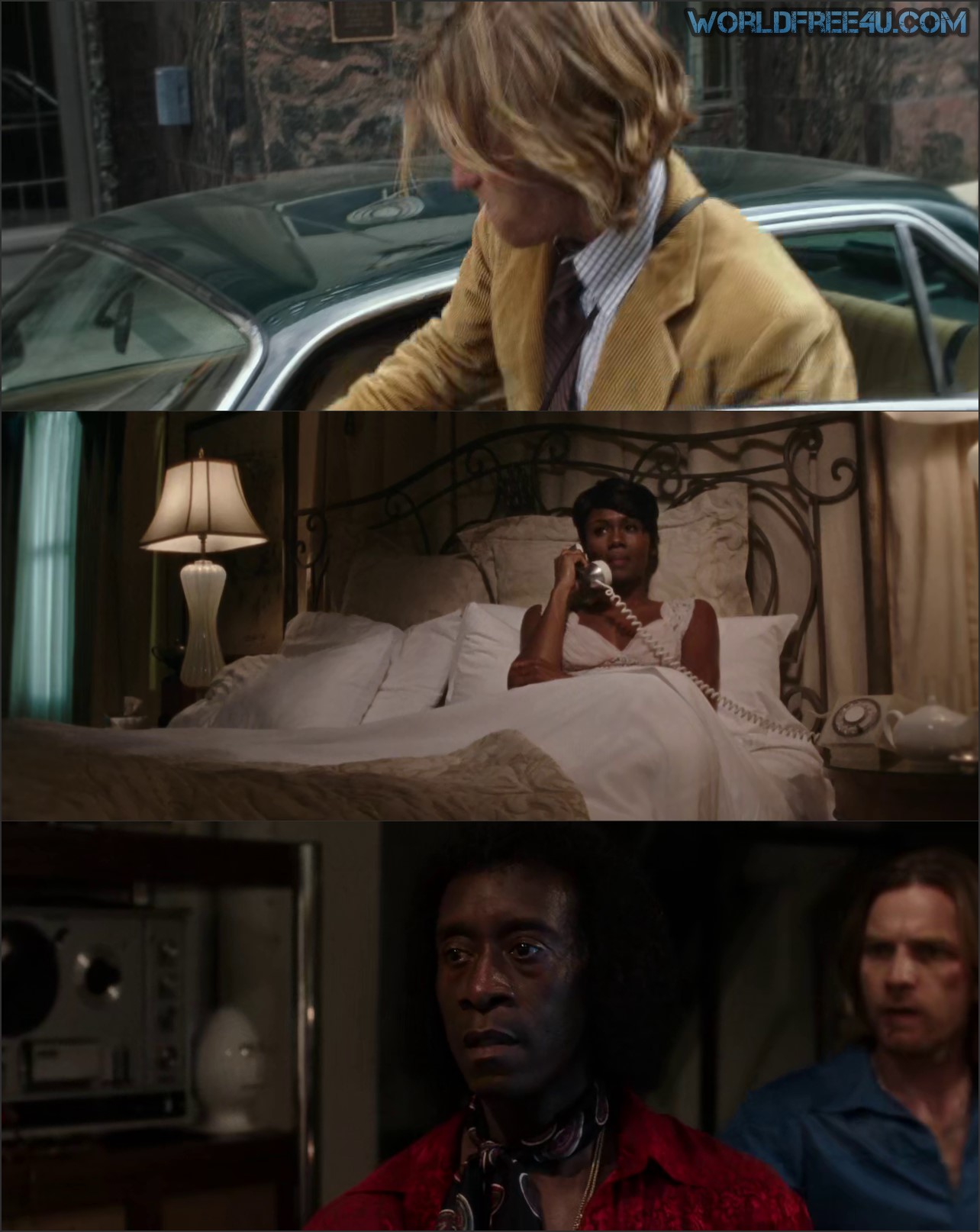This portrait-oriented image is divided into three horizontal sections, each depicting distinct scenes that appear to be from a movie or television show. 

The top section features a Caucasian man with long blonde hair wearing a beige suit jacket over a blue and white checked shirt, complemented by a gray tie. He is either entering or exiting a green sedan, with a backdrop of stone walls that suggests an urban street setting.

The middle section portrays a black woman sitting in a bed under white sheets. She has short black hair and is wearing a white nightgown or tan shirt. She is talking on a corded, old-fashioned telephone that sits on a wooden nightstand next to a teapot. The bed is adorned with numerous white pillows, and there is a transparent or white lamp on the left-hand side, alongside blue curtains.

The bottom section shows a black man with an afro wearing a red, velvety collared shirt and a black and white or black and purple scarf. He stands in the foreground, turning to look toward the left side of the frame. Next to him is a Caucasian man with brown hair, clad in a blue shirt with an open collar. They are positioned in front of a shelf holding some electronic equipment and a white, egg-like object. In the upper-right corner of the image is blue text that reads "worldfreeforyou.com".